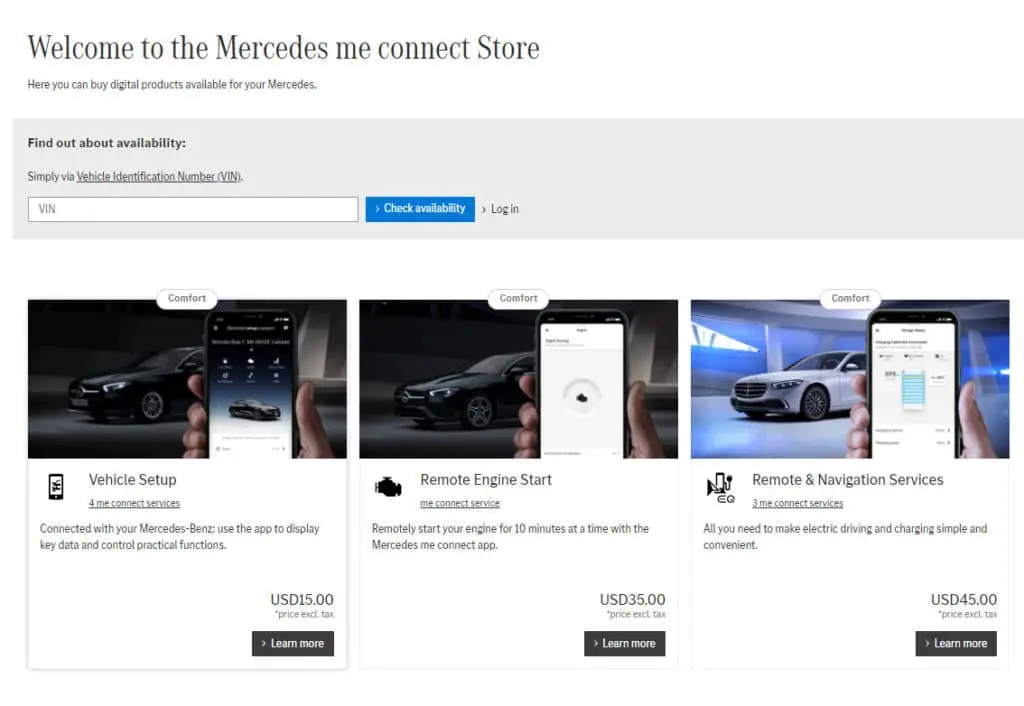**Caption:**

The screenshot showcases various purchase options available on the *Mercedes me connect* store. At the top, a welcoming message reads "Welcome to the Mercedes me connect store," followed by a note that users can buy digital products for their Mercedes vehicles. There is a search field for a Vehicle Identification Number (VIN) to check specific product availability, with a "Check Availability" button located to the right of the search box.

Displayed are three different product options: 
1. **Vehicle Setup - $15:** This feature allows you to connect your Mercedes-Benz to the app, enabling the display of key data and control of practical functions.
2. **Remote Engine Start - $35:** This option lets you start your engine remotely for up to 10 minutes using the Mercedes me connect app.
3. **Remote and Navigation Services - $45:** This service simplifies electric driving and charging, providing all necessary features in a convenient package.

Each option includes an estimated tax and features a dark gray "Learn More" button for additional information. These are categorized under "Comfort Options," distinct from potential economy alternatives.